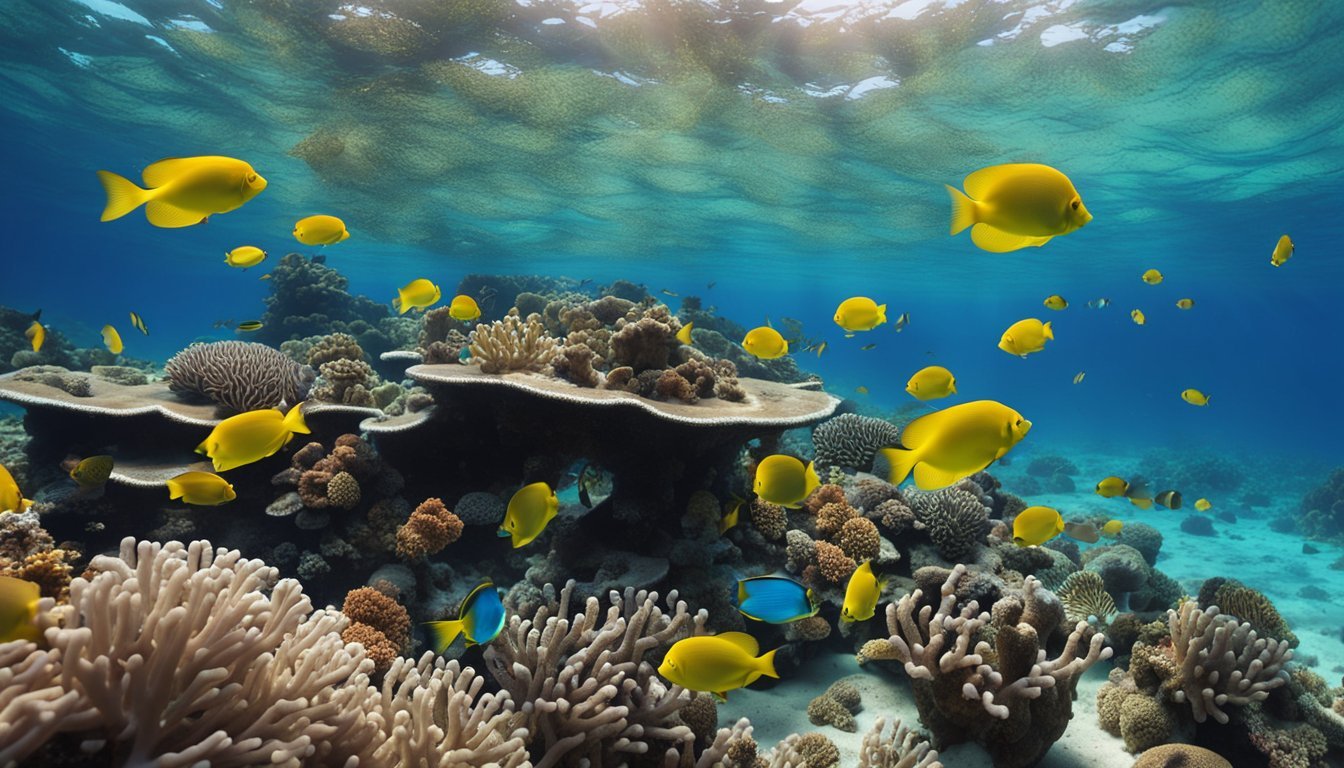This underwater photograph captures a mesmerizing landscape view of the ocean floor teeming with life. The seabed is adorned with an array of corals varying in hues from soft gray to vivid pink and orange, showcasing the ocean's diverse palette. Scattered amidst the corals are numerous oval-shaped fish, all clad in a striking yellow, swimming gracefully through the scene. The ocean's bright blue expanse above fades gently as sunlight pierces through the water, creating a magical interplay of light and reflection that bathes the scene in a serene glow. This serene underwater tableau invites viewers into the tranquil yet vibrant world beneath the sea.